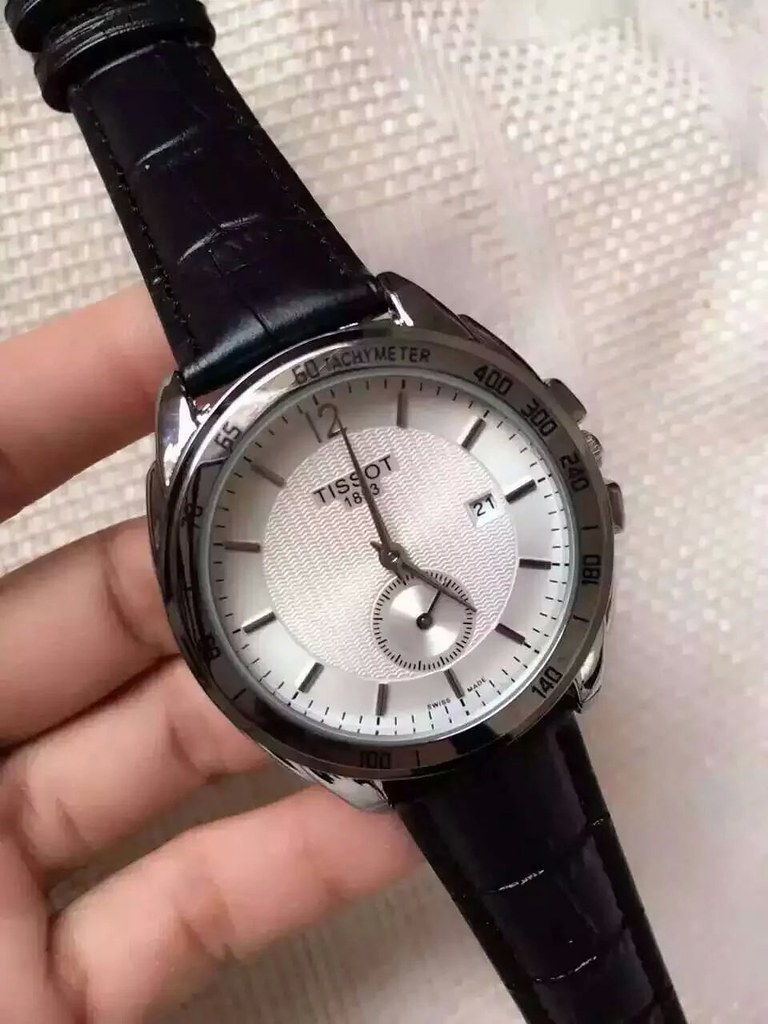In this photograph, a person's hand with light skin is prominently featured. The hand displays visible wrinkles on the fingers, adding a sense of texture and age. The person is holding a sleek, black and silver wristwatch above a white surface that is adorned with fine, tiny circular details. The wristwatch has a black wristband with intricate black stitching that adds to its refined appearance. The clock face is predominantly white, with the singular numeral "12" at the top, accompanied by minimalist silver dashes in place of the other numbers. A polished silver ring encircles the clock face, marked with additional numbers. On the white clock face, the brand name "TISSOT" is elegantly printed in black font, along with some smaller numbers beneath it. The watch's hands are a striking silver, complementing the overall sophisticated design of the timepiece.